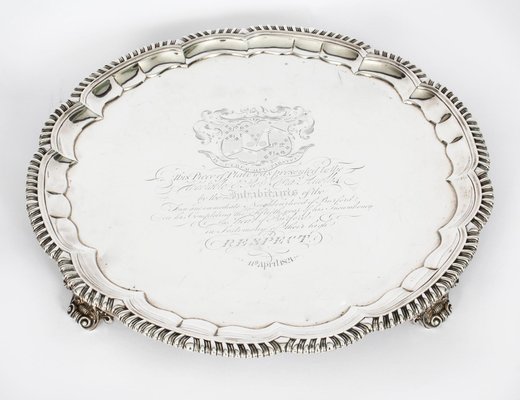The photograph depicts an ornate, silver serving platter with a pair of sturdy but tarnished legs. The platter has a circular, intricate design with ridges and finger-like indentations around the outer border. The central area of the platter is smooth, featuring an emblematic design that seems to resemble a crest or shield, possibly including a heart and ribbon motifs. This emblem, along with an extensive paragraph of text in cursive, is engraved in the middle of the platter. The text appears to be elusive, perhaps even in a language not easily identifiable. The background of the image is a flat gray, providing a neutral backdrop that accentuates the detailed craftsmanship and the contrast between the darker silver lines and the polished silver surface of the platter.